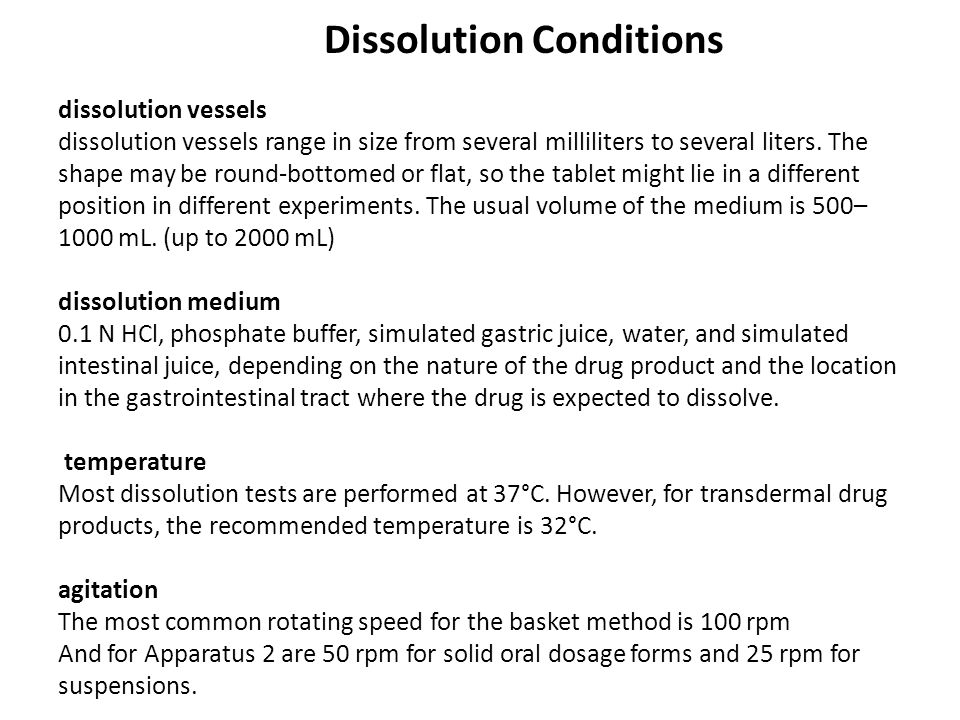The image features a black and white text layout on a plain white background. Entitled "Dissolution Conditions" at the top, the image details various parameters related to dissolution vessels and media used in experiments. The vessels range in size from several milliliters to several liters and can possess either a round bottom or a flat bottom, causing tablets to lie in different positions depending on the experiment. The text specifies that the typical volume of the medium used in these experiments is between 500 to 1,000 milliliters, but it can go up to 2,000 milliliters. It lists various dissolution media, including 0.1 NHCl, phosphate buffer, simulated gastric juice, water, and simulated intestinal juice, chosen based on the drug's properties and the target location within the gastrointestinal tract.

Temperature conditions are also detailed, with most dissolution tests conducted at 37°C, though transdermal drug products are tested at 32°C. Additionally, agitation parameters are mentioned with common rotating speeds for different methods: 100 RPM for the basket method, 50 RPM for apparatus 2 in solid oral dosage forms, and 25 RPM for suspensions. The text is neatly spaced, well-organized, and suggests a digital or print format, possibly from a PowerPoint presentation.